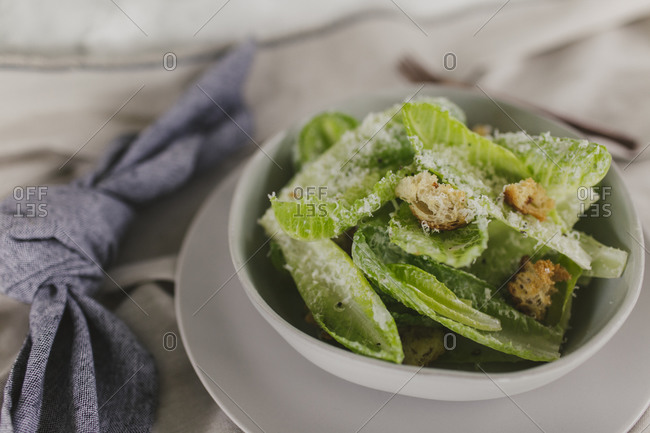The image is a close-up stock photo of a small, simple salad in a white ceramic bowl, placed on a white ceramic plate. The plate and bowl are positioned in the lower right-hand corner of the frame, taking up most of that portion of the image. The salad consists of some type of greens, likely spinach or kale, lightly dusted with finely shredded parmesan cheese and sprinkled with a few small croutons. The entire setup is sitting on a whitish-gray tablecloth, with visible rumples. To the left of the plate, there is a light blue napkin twisted into a knot. A blurry fork is positioned behind the plate. Additionally, the image features a subtle diagonal watermark with offset letters including "O" or possibly a zero, typical of stock photos. The overall scene suggests a restaurant setting.